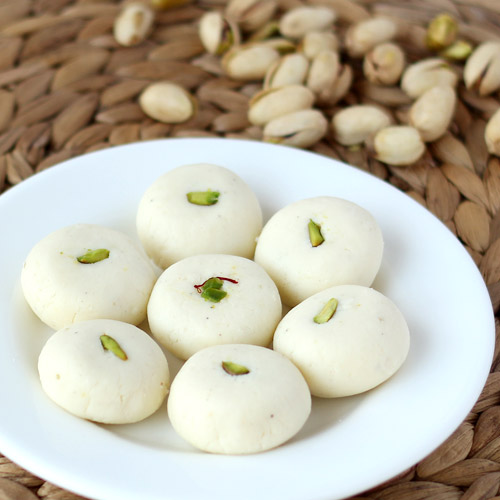The image features a white plate resting on a woven rattan placemat, showcasing seven round, dessert-like items possibly resembling mochi or cookies. These items are arranged in a flower-like formation with six positioned in a circle around one in the center. Each treat is primarily white or beige in color and is topped with what appears to be a piece of pistachio nut. This is reinforced by the presence of empty pistachio shells visible in the background. The treats have a flat, biscuit-like appearance, and their precise identity is not stated. The overall presentation is clean and simple, emphasizing the contrast between the white plate, the light-colored desserts, and the green pistachio pieces.